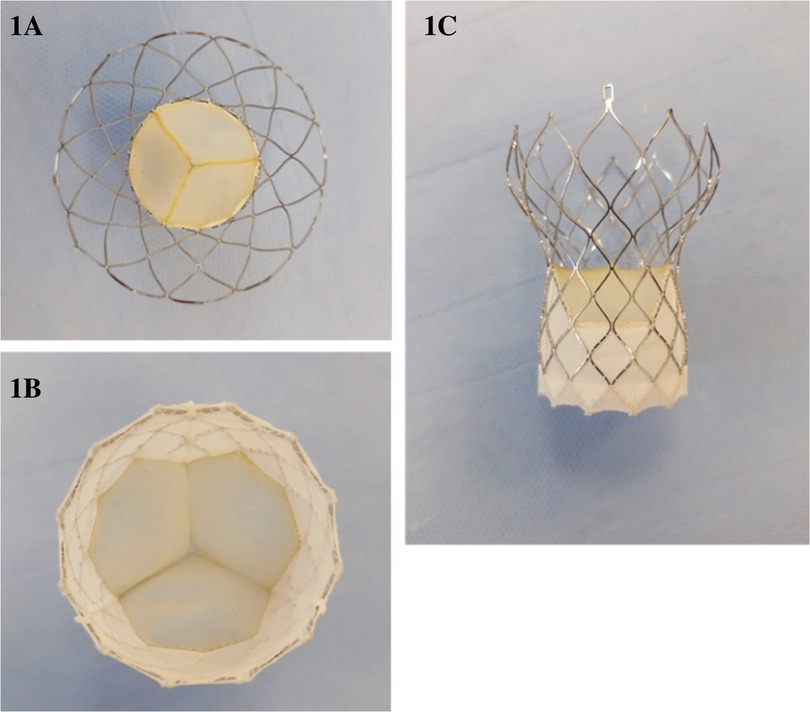The image displays a detailed examination of a decorative object, potentially a lantern or candle holder, through three distinct labeled views—1A, 1B, and 1C—arranged against a gray surface. 

1A offers an aerial perspective of the object, revealing a three-piece circular design with intricate metal wiring around the top. This view highlights a central component with a white and yellowish hue, suggesting a spherical or cylindrical shape.

1B provides an internal look directly into the hollow cylinder, exposing the outline of the same metal wiring seen in 1A, but from the inside. The transparency of this part adds to the object’s holographic appearance.

1C presents the side view, showing how all components fit together. This perspective clearly illustrates the shape and structure of the assembled object, with the hollow tube and overlaid metal design. A hook on one side implies that the object can be hung, indicating potential use as a hanging decoration. The background in all images features a consistent light gray to light blue gradient, enhancing the visibility of the detailed design.